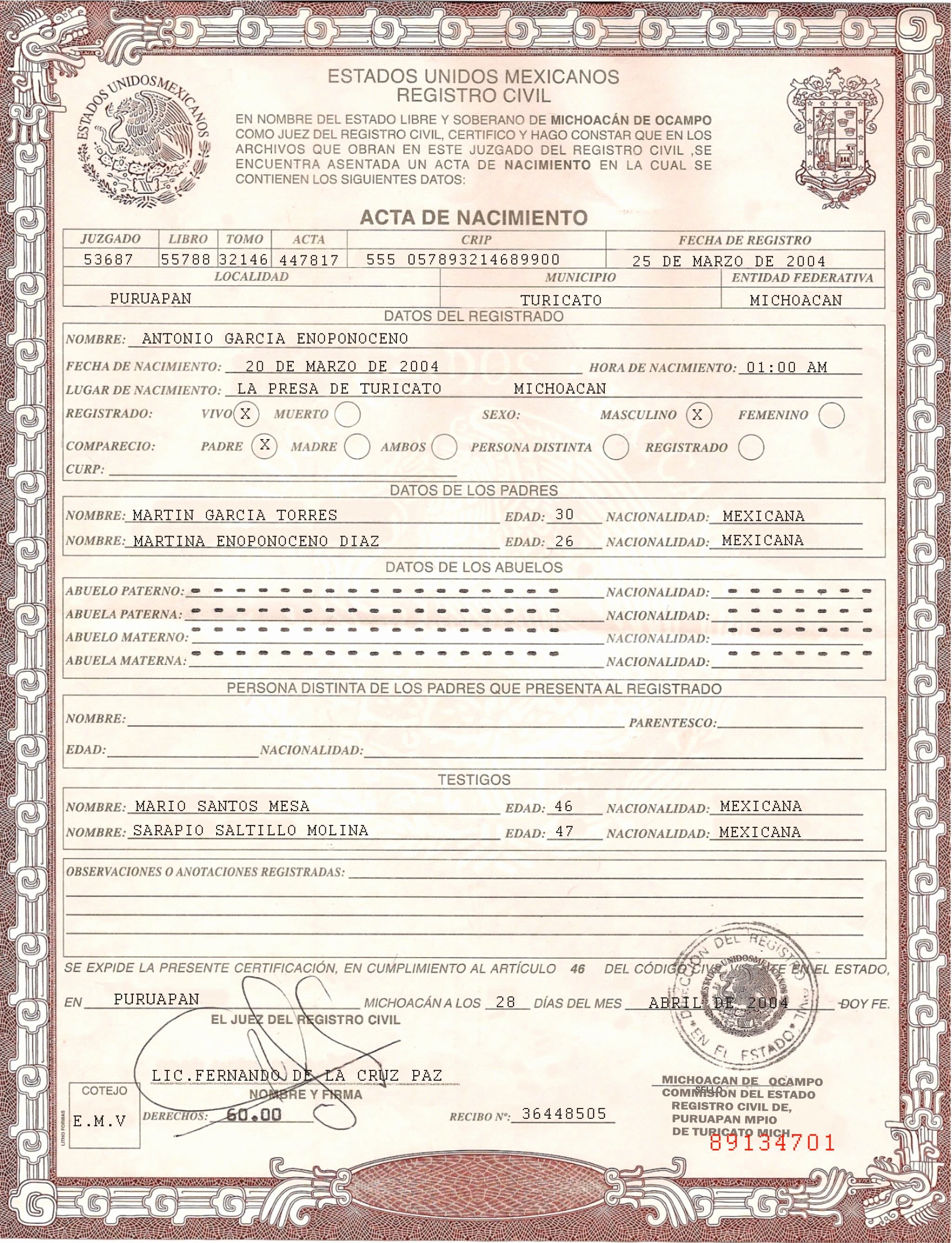The image depicts a scanned legal document from Mexico, showcasing a detailed and ornate design in brown and white hues. At the top, the text "Estados Unidos Mexicanos Registro Civil" identifies it as an official civil registry document, likely a birth certificate. The document's border features an intricate illustrated dragon extending all the way around. The form, filled out with a typewriter, has several sections. The "Nacimiento" section is followed by a table filled with details including a name, date, and time of birth, identified as Mario San Pio's Mesa and Garfield Antillo Molina. Below this, another section labeled "Datos de los Padres" lists the nationality and names of the parents, confirming their Mexican origin. The lower portions of the form remain blank, but there's a signature at the bottom left, alongside a slightly faded stamp and a prominent red number, 89134701. The document also bears seals, adding to its authenticity. The style and layout are indicative of a mid-2000s issuance, suggested by the specificity of the date being around 2004.